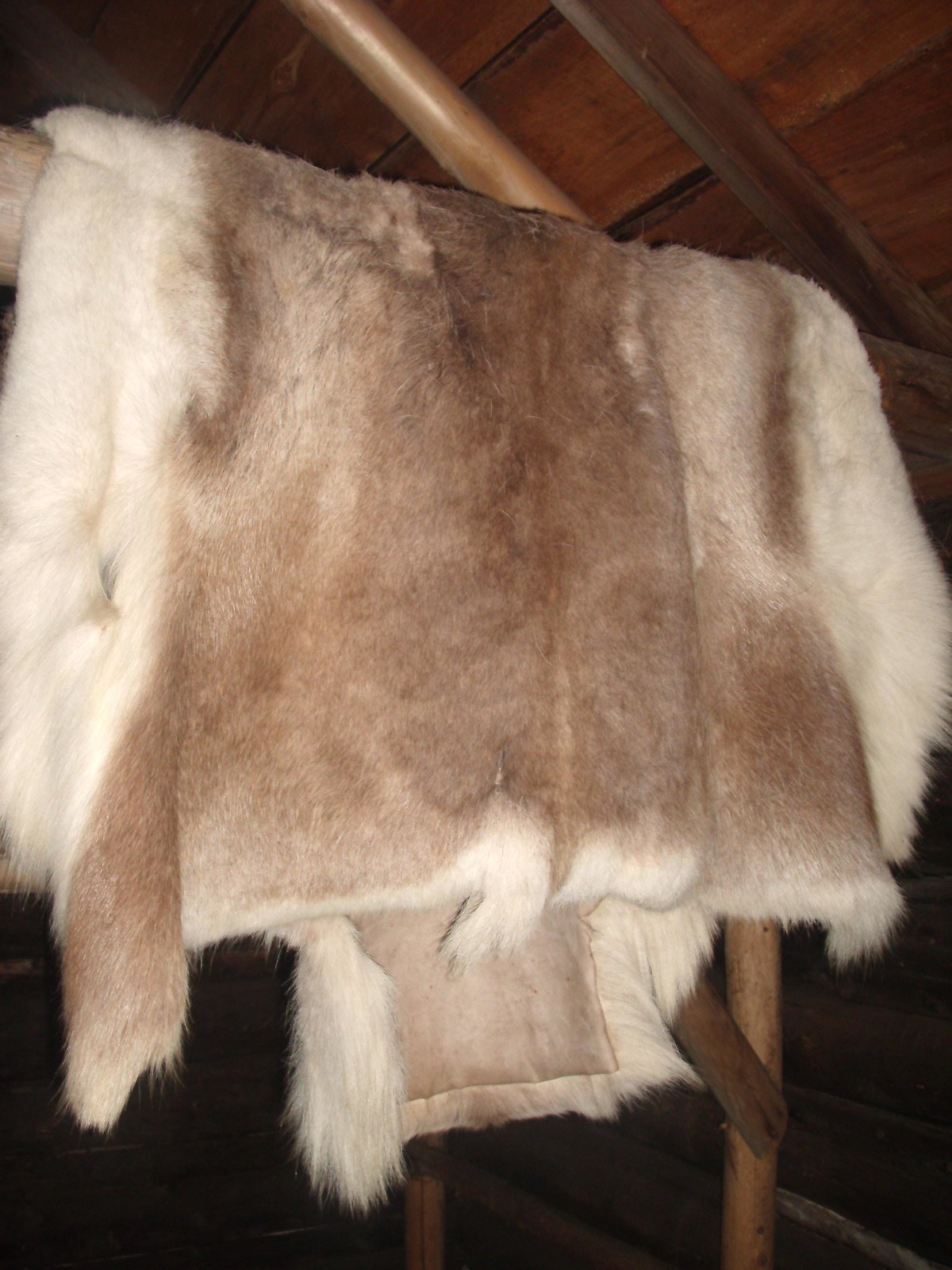The image depicts an animal hide with soft, fluffy fur, displayed inside a wooden structure that resembles a barn or rustic building. The hide, which is predominantly tan in the center and transitions to white on the edges, is folded over a wooden pole, revealing only half of it. The tips of the fur, particularly in the front, feature longer pieces that hang down, including a noticeable brown piece on the left and a small white tuft in the center. The inner side of the pelt shows the leather backing to which the fur is attached. The ceiling of the room is visible in the background, showcasing dark wooden rafters arranged in intersecting patterns. The pole that supports the hide appears to be part of a nailed-together structure, although the full extent of this support is not visible due to the close-up nature of the image.